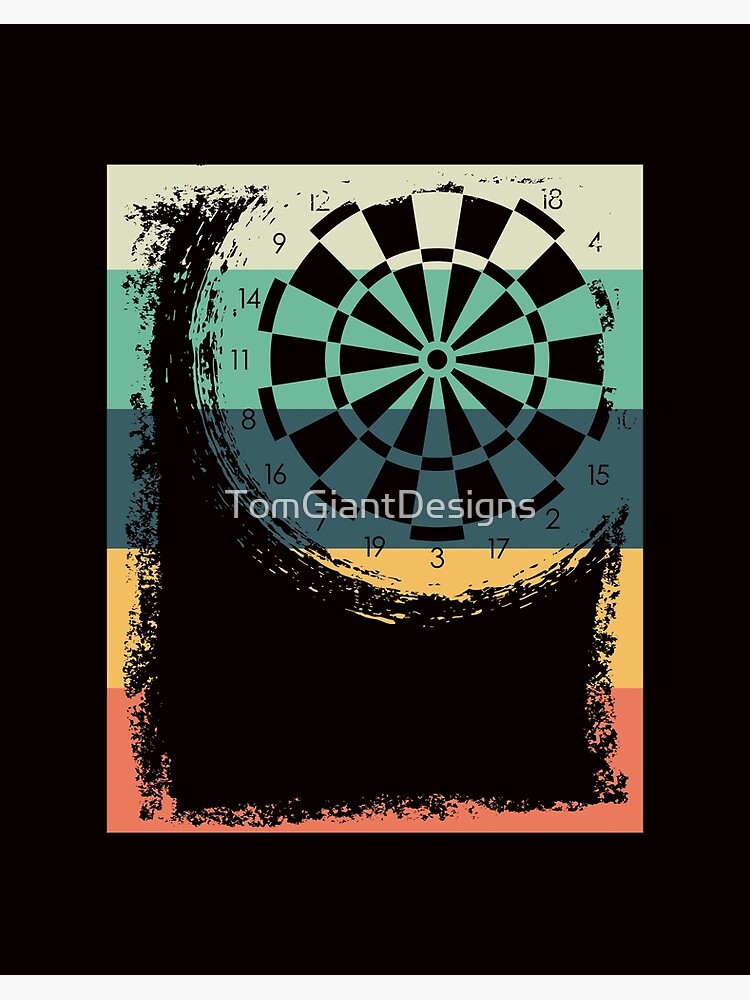The image, a vertical rectangular computer-generated poster, advertises "Tom Giant Designs" with the text prominently displayed in white letters in the center. The background is primarily black, but there is a smaller rectangle within it featuring horizontal stripes in white, green, blue, yellow, and orange from top to bottom. A black abstract design with fuzzy edges overlays the bottom part of the striped rectangle. Positioned centrally within this black overlay is a distinctive, circular dartboard design, complete with a black center, recognizable triangular shapes, inner and outer rings, and numbers including 3, 19, 17, 7, and 2. The dartboard’s pattern integrates seamlessly with the layered colors and abstract design, creating a dynamic visual effect.